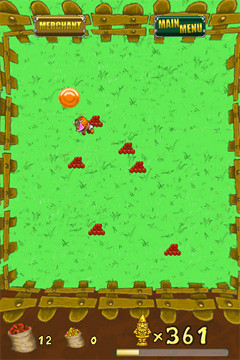The image appears to be a screenshot from a video game interface. The screen predominantly features a green background, bordered by what resembles brown painted picket fencing along the top left and right edges. This gives the scene a rustic, garden-like ambiance. At the bottom of the screen, there is a brown border that contains player information displayed in yellow text.

Towards the top of the green area, a gold coin is visibly placed, adding a touch of treasure-hunting allure. Interspersed within the scenery are clusters of red berries or fruit, providing a splash of vibrant color. A small, purple character stands out in the foreground, notable for its orange hair and feet, along with some red detailing on its face.

In the top left corner, the word "Merchant" is prominently displayed in gold letters, indicating a possible in-game vendor or shop. To the right, the phrase "Main Menu" appears in gold letters as well, set against a green background, suggesting navigational options for the player.